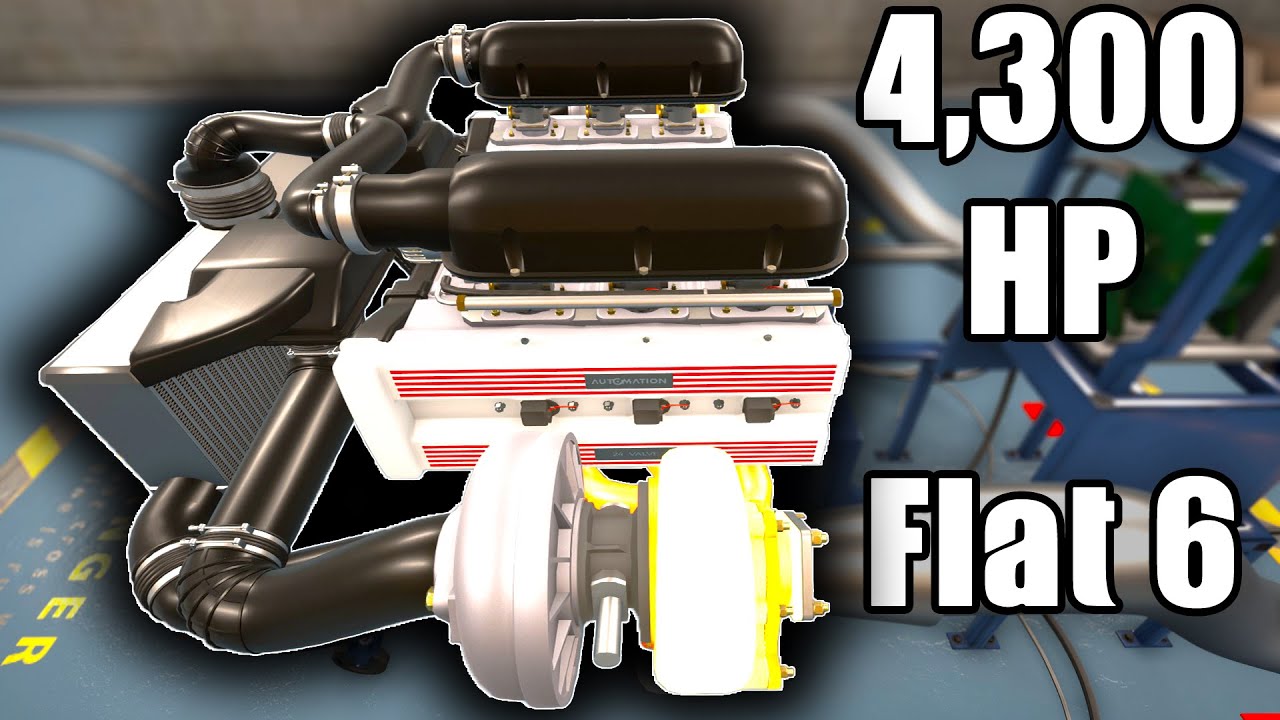The image is a highly detailed, stylized graphic of a car engine, prominently featuring a 43 HP flat-six cylinder configuration. White text on the right side of the image reads "43 horsepower flat 6," bordered with a black outline. The engine is displayed in a technical, diagram-like manner, with most of the lines rendered in black and the engine block itself in white. Red-striped lines extend across the engine block, accentuating its contours, with charcoal-colored buttons visible on the side.

The engine includes identifiable components such as gray fuel filters, a gas cap, an air filter, and a radiator. The black plastic piping snakes over the engine block, further enhancing the technicality. There's also a turbo-like snail and an intercooler, suggesting a complex setup possibly linked with an intake system. The foreground features white or powder-coated valve covers with ignition plugs seated on the cover head.

In the background, the engine is photoshopped against a blur of steel-like, dark blue painted surfaces with hints of silver piping, yellow text, and indistinct blue hues. This creates a metallic, industrial aesthetic, making the engine's details pop even more. The entire composition seems to be a video thumbnail, presenting the engine as though it's mounted in a stationary setup, casting a black glow around it for added emphasis.